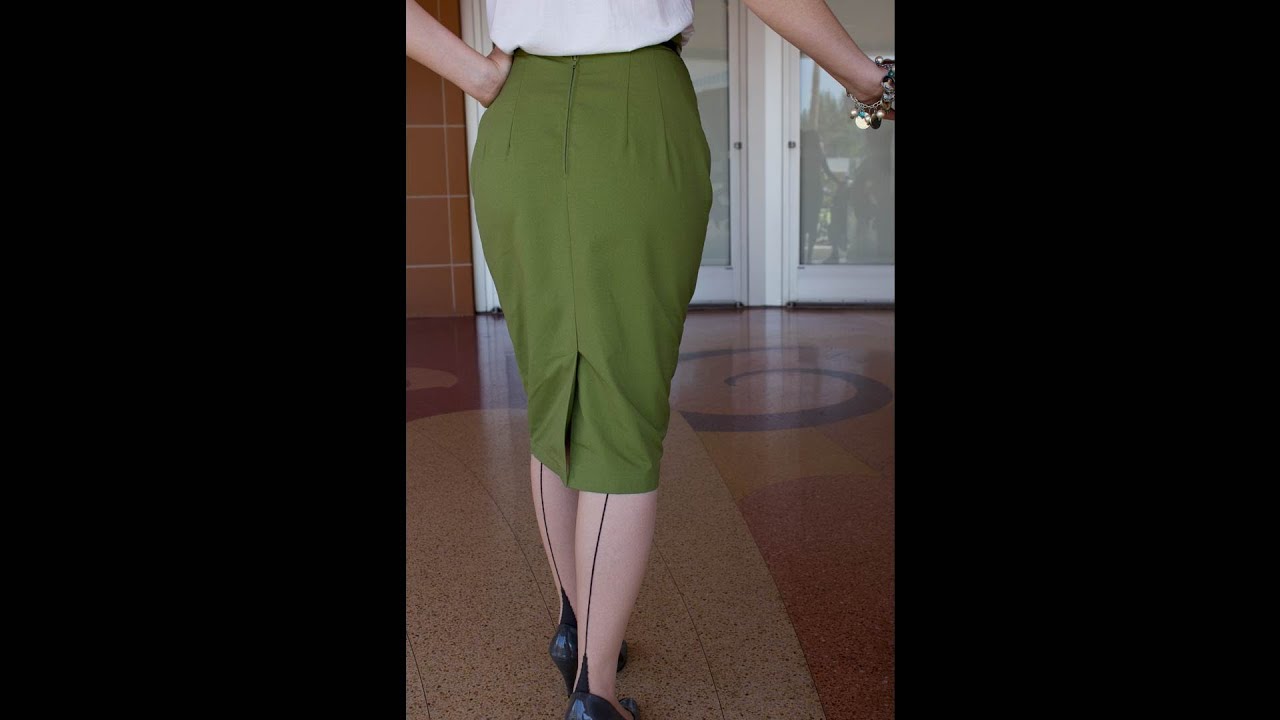The image is a detailed color photograph in portrait orientation, showcasing the backside of a slender woman of likely Caucasian descent. Her attire consists of a fitted, light green pencil skirt that extends below her knees, featuring a pleat at the back, and a white blouse. Her legs are clad in transparent stockings with distinctive black seams running vertically up the back. She stands poised in black heels on a granite floor with a brownish-reddish hue. One of her hands is sitting confidently on her waist, while the other rests on an unseen object or surface. Her right wrist is adorned with shiny, silver charm bracelets. The indoor setting includes a white door in the background and walls lined with brown square tiles, suggesting a commercial foyer or the entrance of a building. The image captures her from just above the waist to the floor, emphasizing representational realism.